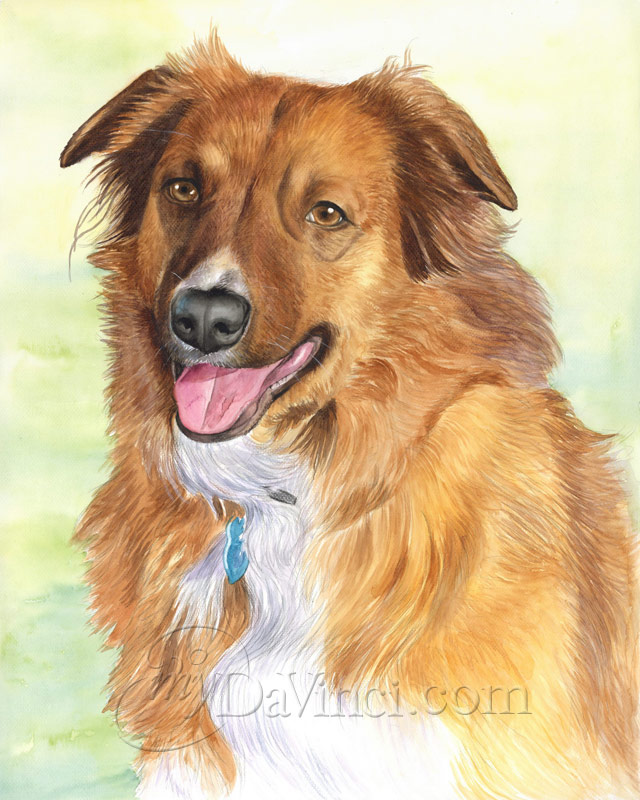This highly detailed and realistic painting features a beautiful, fluffy medium-to-large dog, resembling a collie mixed with a German Shepherd. The dog sports a rich, golden brown coat with tan, brown, and white accents, including a prominent white chest and underbelly. Its soulful brown eyes, black nose, and pink tongue add to its lifelike quality. The dog's ears flop slightly, and it wears a blue collar tag around its neck. The background of the painting is a blend of green and blue, slightly blurred to draw focus to the dog, and the artwork is marked with a watermark reading "DaVinci.com" at the bottom. The dog is captured in a vertical image, panting gently, giving a touch of warmth and personality.